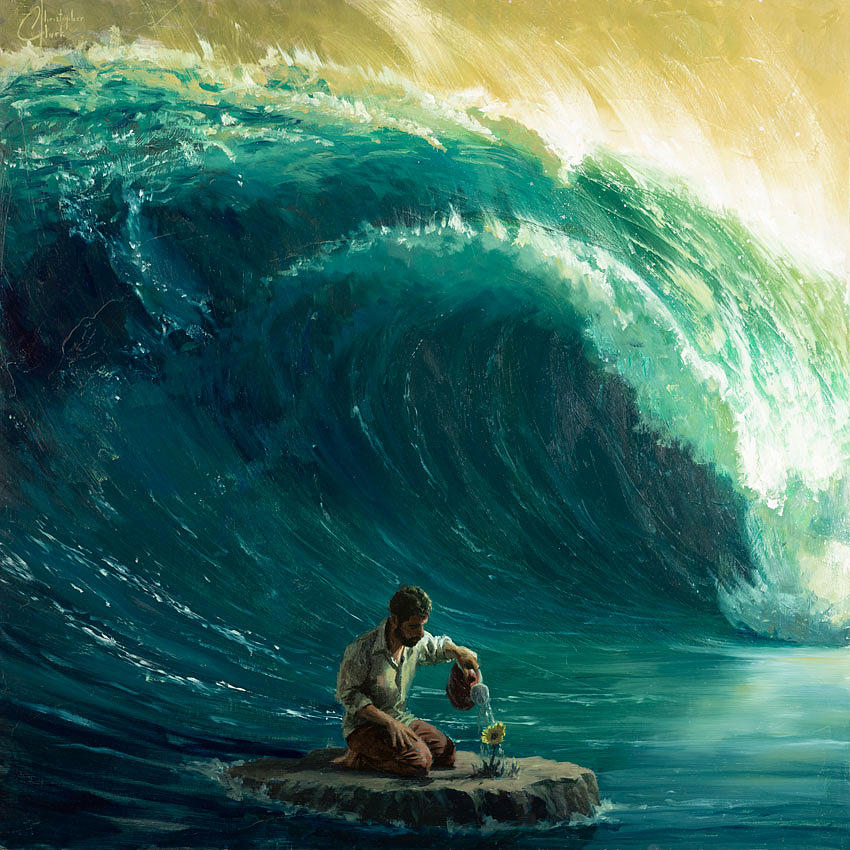In this vivid painting, a man with short dark hair, clad in a collared shirt and brown pants, is depicted standing on a large rock that forms a tiny island in the middle of a vast, tumultuous ocean. This rock barely accommodates him as he kneels down, tenderly watering a delicate yellow flower emerging from the rough surface. Surrounding him, immense blue-green waves, painted with intricate detail, rise menacingly in the background, poised to crash down with their formidable power, their heights towering two to three times above him. The sunlight illuminates the scene, adding a bright yellow hue to the sky, which contrasts dramatically with the dark, frothy waves. This striking image captures the quiet act of nurturing life amidst overwhelming natural forces, set against a brilliantly defined, sunlit seascape.